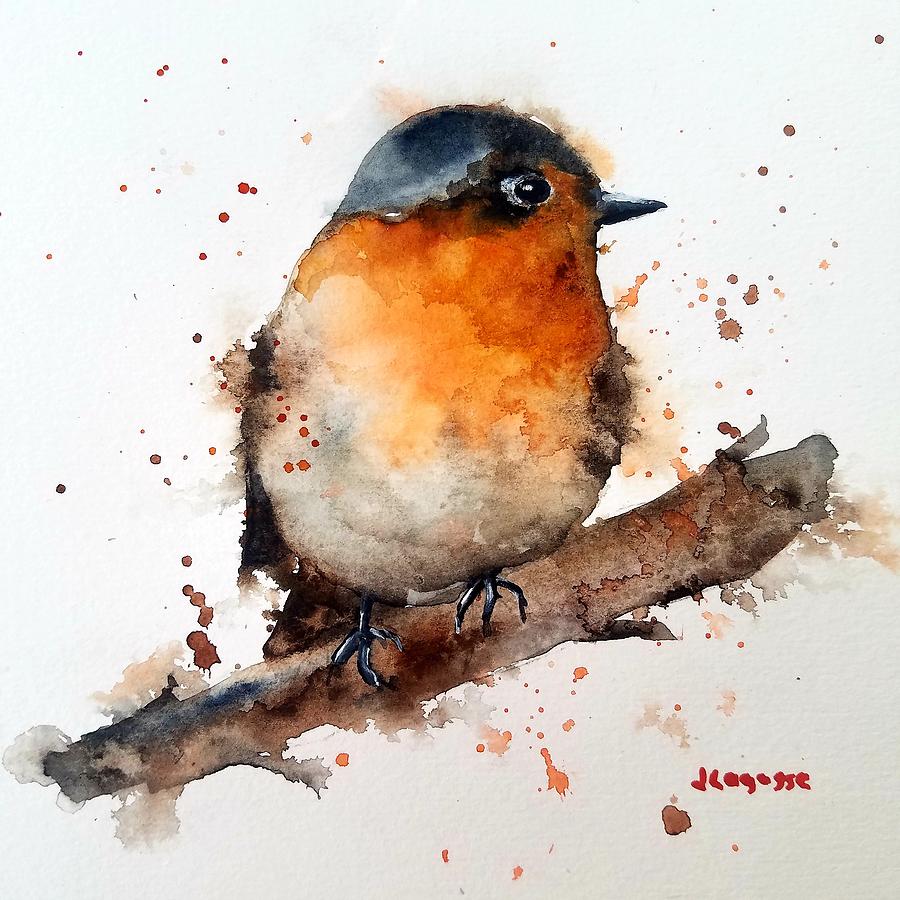This is a detailed watercolor illustration of a small, slightly chubby bird perched on a branch. The bird features a black head, a short pointed black beak, and white ringed eyes with a central black dot, adding a lifelike touch. It has an orange neck and chest, transitioning into a lighter orange and white belly. The bird’s black and brown wings and brown tail feathers give it a distinct appearance. Its small black legs grip a brown branch with tinges of black and gray, extending diagonally from the lower left to the middle right of the painting. The background is a textured, gradient canvas that fades from bright white in the upper left to an off-white in the lower right. The artwork has an impressionistic feel, with paint splatters of orange, brown, and red around the bird, enhancing the vivid scene. A small, red signature sits in the lower right corner.